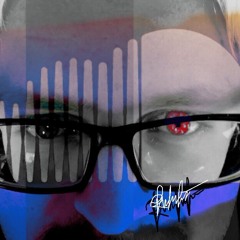This black-and-white close-up image features a blonde man wearing prominent black Buddy Holly or Elvis Costello horn-rimmed glasses. One of his eyes is strikingly red, possibly due to a colored contact lens, while the other eye appears dark or black. The lower portion of the image, especially around his nose and cheek, is washed in a blue transparent color that adds a comb-like graphic design layer. The blue extends from the bottom part of the image up to one of his eyes. There is a small, illegible signature across his face, adding to the artwork's enigmatic quality. The overall aesthetic suggests the look of a stylized album cover, though the identity it advertises is unclear. The image's composition, with its bold use of color and close-up facial focus, delivers a visually striking and somewhat surreal presentation.